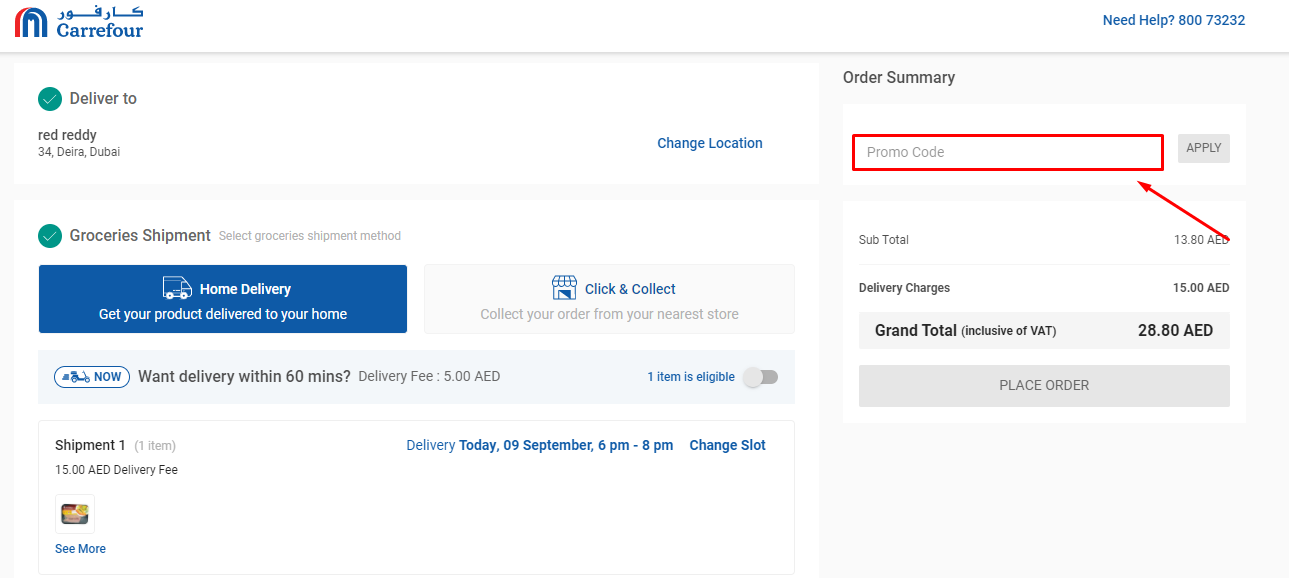**Descriptive Caption:**

The screenshot displays a web page with a white background. At the top of the page, there is a logo consisting of two blue arches with a red arch extending to the side. Adjacent to the logo, non-English characters are visible, possibly Hebrew or Arabic, and directly beneath it, the word "CARREFOUR" is spelled out. To the right of the heading, there is a prompt that says "Need Help?" followed by the phone number 800-732-32. 

Below this, a grey line separates the header from the main content. Directly underneath the grey line, the text "Deliver To" appears, followed by a green circle with a checkmark symbol and the address "34 DEIRA DUBAI" in red text. To the right of this section, there is the option to "Change Location."

Further down, there is a section titled "Groceries Shipment" where users can select their shipment method. The options available are "Home Delivery" with the description "Get Your Product Delivered To Your Home" and "Click and Collect" with the description "Collect Your Order From Your Nearest Store." The "Home Delivery" option is currently selected.

Beneath this, the page displays a special option for expedited delivery: "Want Delivery Within 60 Minutes" with a delivery fee of 5 AED, noting that one item is eligible for this service. The standard shipment section follows, labeled "Shipment 1," which has a 15 AED delivery fee and is scheduled for "Today 09:00-10:00 PM" with an option to change the delivery slot.

On the right-hand side of the page, there's a section for entering a promo code, along with a summary of the cart totals. The subtotal is listed as 1380 AED, with an additional delivery charge of 15 AED, bringing the grand total to 28.80 AED.